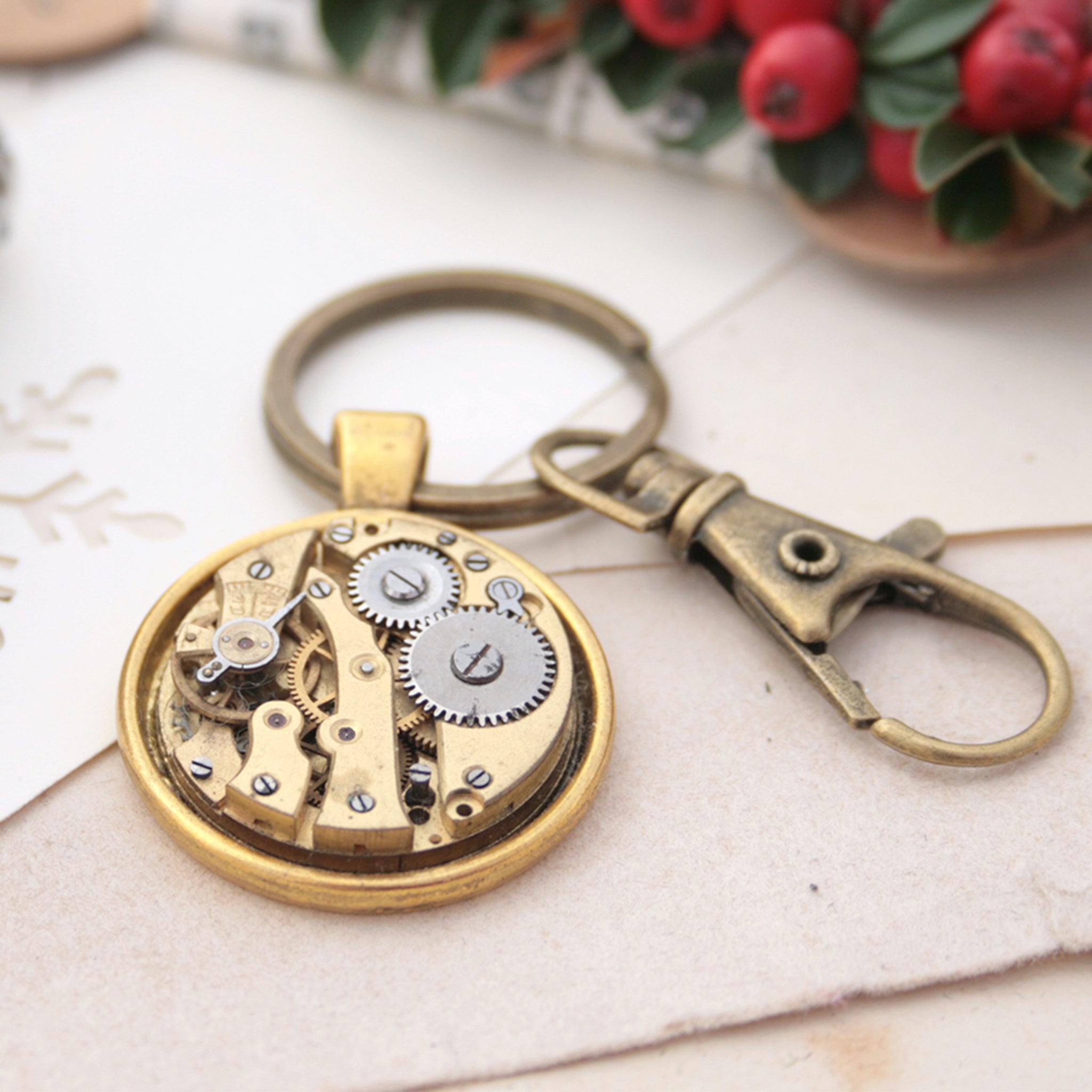The photograph showcases a steampunk-inspired keychain laid out on a multi-layered, flat surface. The surface includes three pieces of tan construction paper, one piece of white paper with a snowflake cutout, and a small round platter visible in both the top left and top right corners. In the top right corner, there is a cluster of berries attached to a green leafy stem positioned on the platter. Central to the image is the keychain, featuring a round bronze pendant resembling the intricate inner workings of a mechanical watch, complete with exposed silver and gold gears and clockwork components. The pendant is connected to a bronze ring and a clasp, emphasizing its steampunk aesthetic. The overall scene combines elements of mechanical intricacy with a layered, visually rich background.